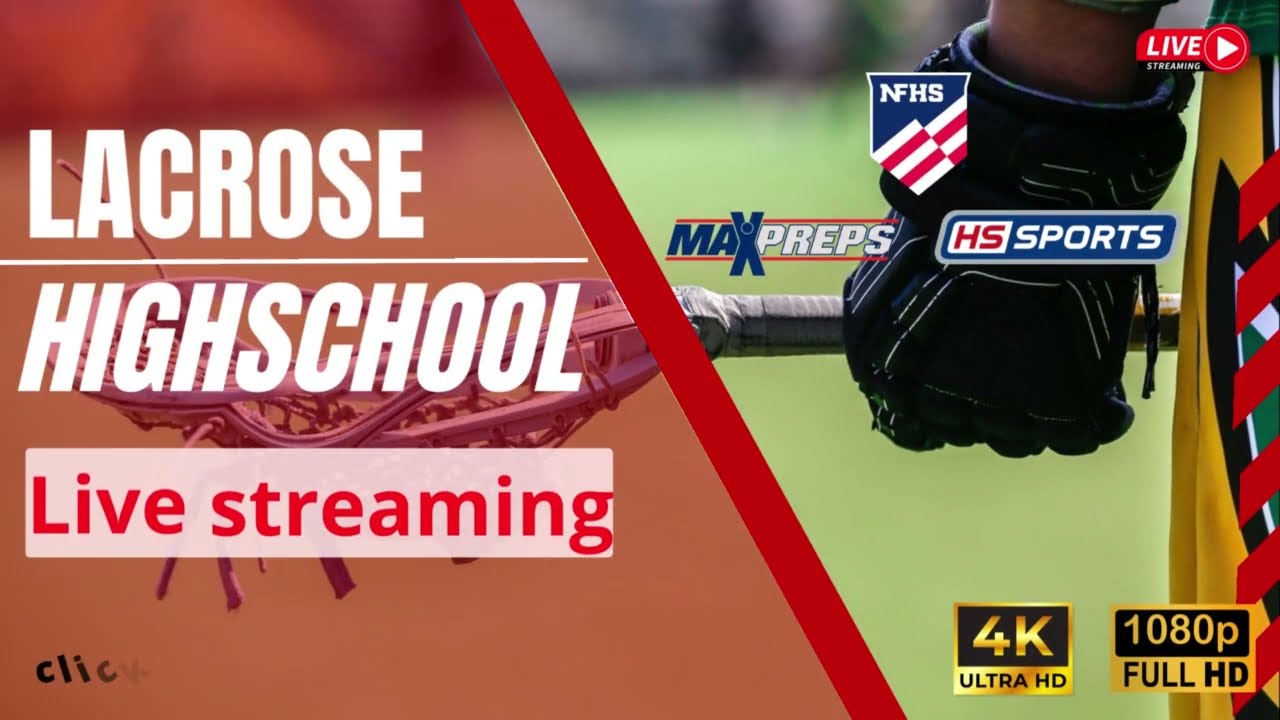This advertisement features a high school lacrosse live stream. The left side of the image has a reddish peach background, transitioning to a red background, with the text "La Crosse High School" in white font. Below this, a white rectangular box contains the words "live streaming" in red, and the term "CLICK" is displayed diagonally in black font. A red diagonal line divides this section from the green background on the right.

The right side portrays a close-up of a lacrosse player’s hand gripping a lacrosse stick, with the stick extending over into the red section. The player is wearing a black glove and yellow shorts with green and white diagonal stripes. At the upper right corner, there's a red rectangle encasing the word "live" with a play button icon. Over the glove area, there are various logos including NFHS in a red, white, and blue shield, MaxPreps, HS Sports, and a marker indicating 4K Ultra HD and 1080p Full HD quality displayed in black and gold font.